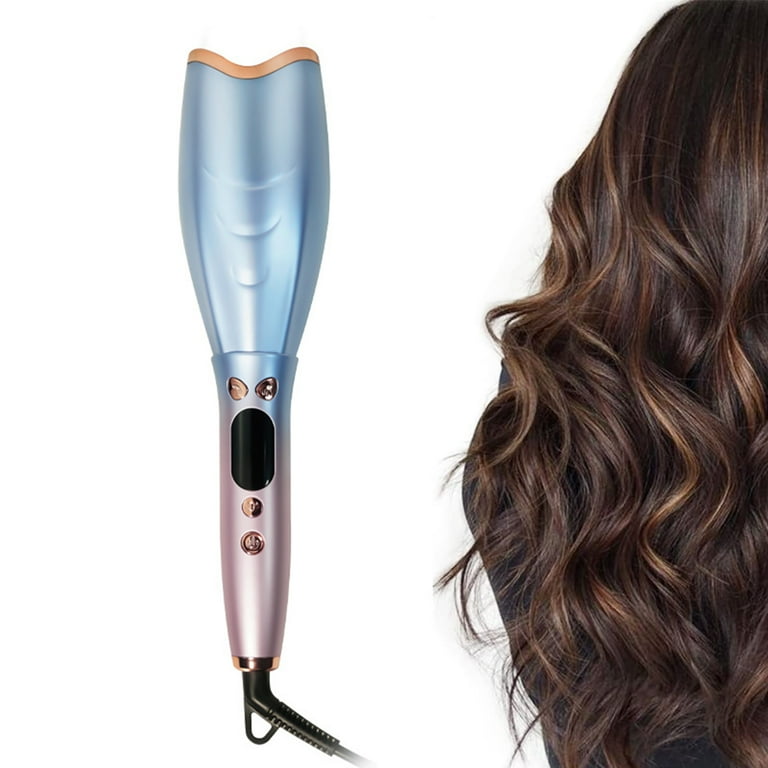The image features an advertisement for a women's hairstyling product against a white background. On the left, there is a sophisticated hair tool that appears to be a hybrid straightener and curler. The device showcases a light blue, tulip-shaped top with gold edging that fades into a rose gold handle. The handle is adorned with four buttons: two small gold ones near the base of the blue section, and two circular rose gold buttons aligned vertically. Additionally, there is an oval-shaped black screen likely meant to display heat settings. The appliance is connected to a black cord, which extends towards the bottom right of the image. To the right of the screen is the back view of a woman’s head displaying long, flowing, wavy brown hair with subtle caramel highlights, suggesting the effectiveness of the styling tool shown.